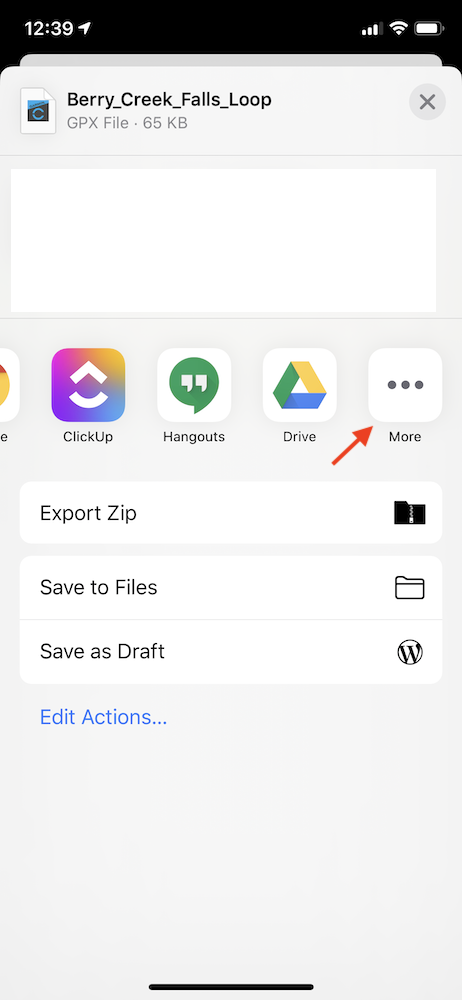### Description:  
A detailed view of an admin panel interface displayed on a smartphone screen at the time 12:39, with three to four bars of signal strength, full Wi-Fi connectivity, and approximately 90% battery life, all visible on a black header at the top. Below the black header, there's a gray inset field partially obscured by a pop-up overlay.

The overlay displays the title "berry_creek_falls_loop" at the top. Below the title, there's a GPX file icon on the left, indicating a file size of 65 kilobytes, and a close button on the right. A thin gray line separates this section from the rest of the overlay content.

In the central section, several app icons are visible: most of one app on the far left is cut off and unreadable, followed by ClickUp, Hangouts, Drive, and a three-dot icon indicating more options. A red arrow overlays the screen, angled at 45 degrees from the lower left and pointing upward towards these app icons.

Below these icons are three options presented with associated icons on the right:  
1. **Edit, Export, Zip** - associated with a zip file icon.  
2. **Save to Files** - accompanied by a standard file folder icon.  
3. **Save as Draft** - denoted by the WordPress icon (a "W" in a circle).

Further down, a blue text link reads "Edit Actions..." providing an additional layer of options. At the very bottom, a plain black bar is visible, consistent with the design of the device's interface. The rest of the background remains unadorned, emphasizing the administrative functions in focus.